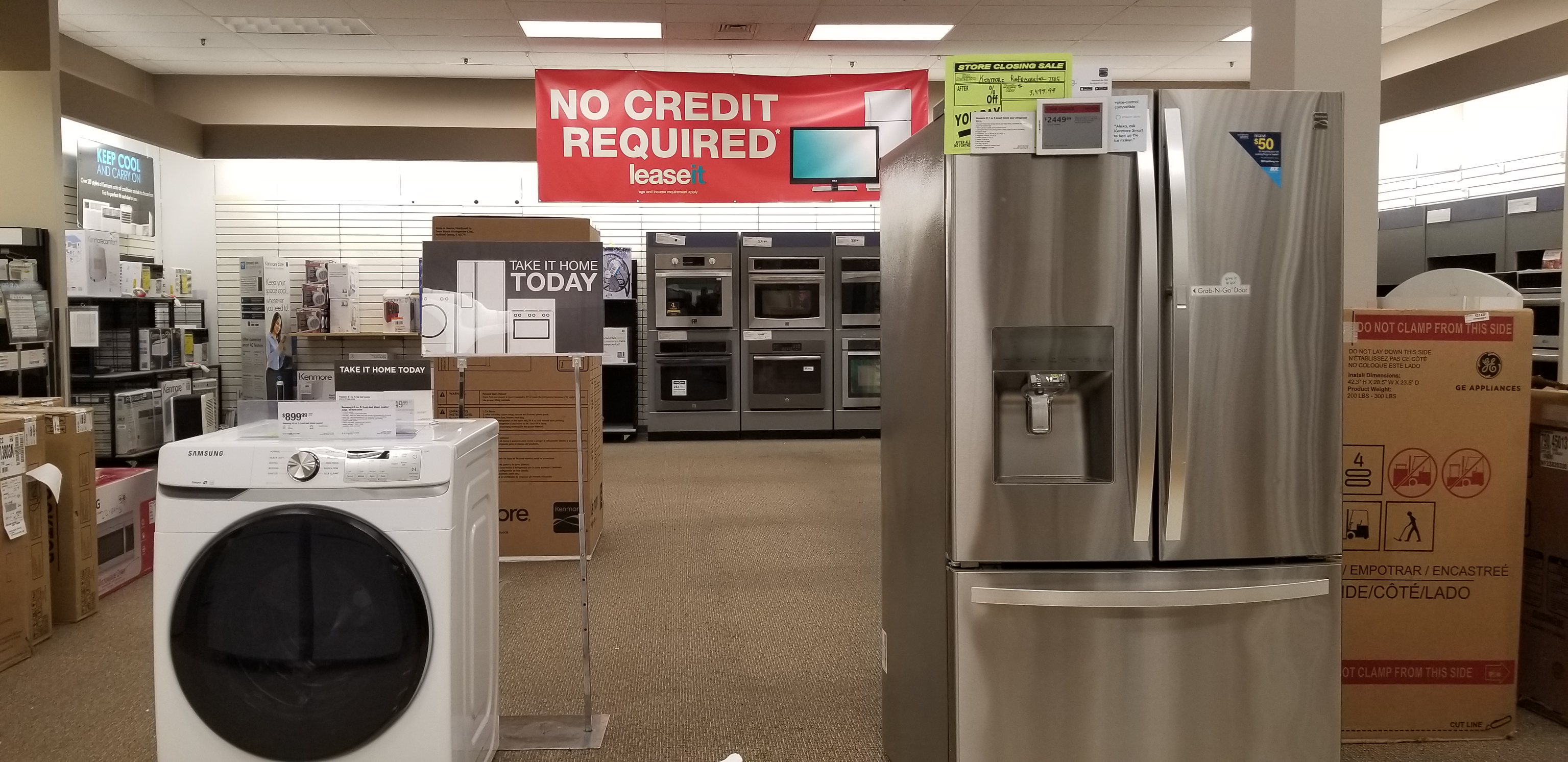This real-life image captures the bustling interior of an appliance store. The central ceiling features a tiled pattern with square lights, and a prominent red banner hangs below, emblazoned with "No Credit Required, Lease It" in white text, except for the blue word "it." Adjacent to the banner is an illustrated television and a white refrigerator. The store's floor is carpeted, and the backdrop reveals an array of stoves or ovens. To the right, partially obscured by a large stainless steel refrigerator, are possibly more ovens. This refrigerator, equipped with a bottom freezer, right-side door, left-side door for the top half, and a water or ice dispenser, bears a small triangle sticker and a cluster of yellowish neon papers and stickers, likely displaying product information and pricing. A cardboard box sits nearby, backed by a store pillar. On the left, a white appliance, possibly a washing machine or dryer with a black-tinted viewing panel, stands beside scattered papers. The left wall is lined with various boxed products, which might include microwaves. A striking black sign in the middle declares "Take it Home Today," set against a backdrop of illustrated household appliances, adding to the vibrant display of the store’s offerings.